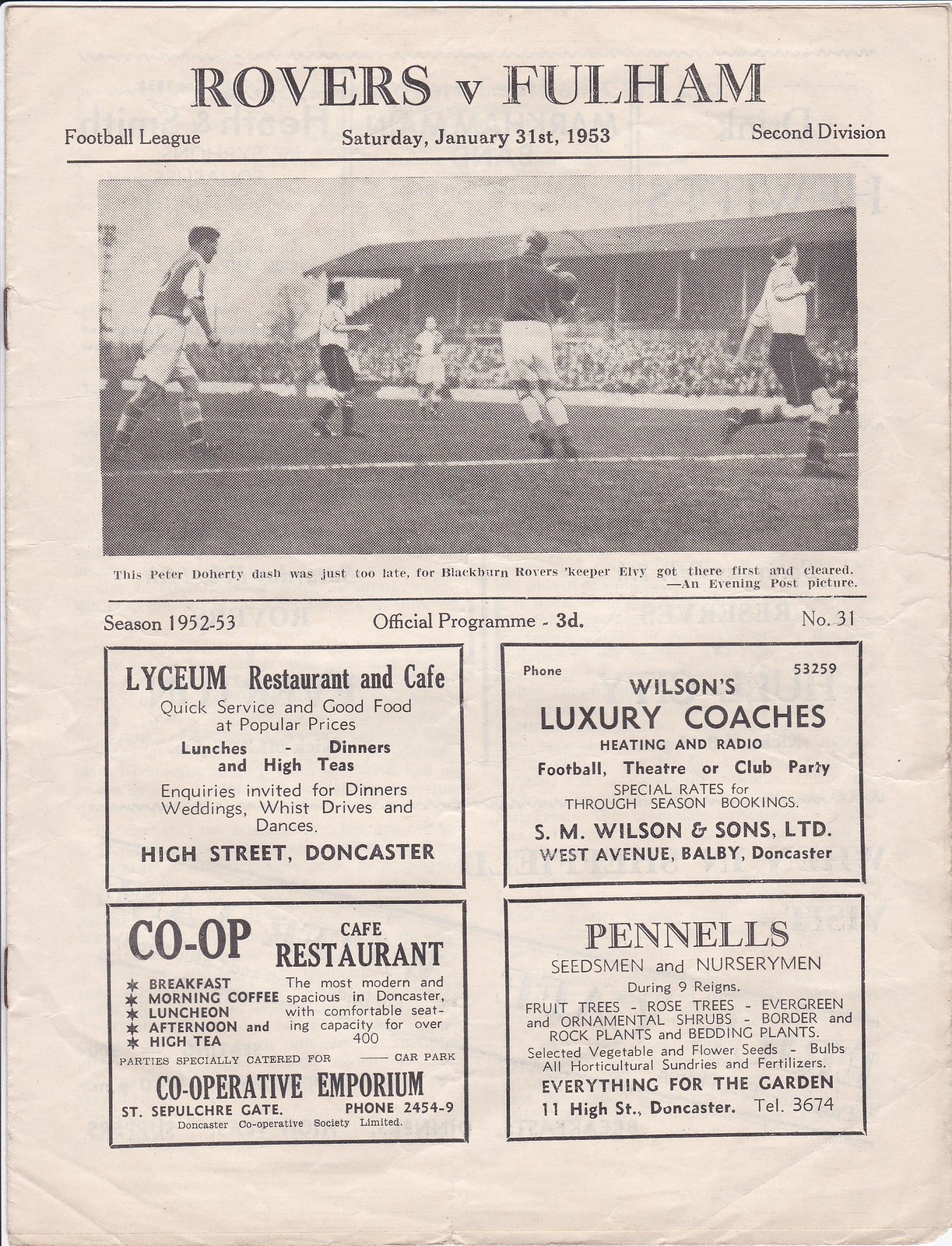The black-and-white image is a page from a newspaper featuring an advertisement at the top under the headline "Rovers v. Fulham" in black lettering. Beneath this, small letters on the left read "Football League," the center states "Saturday, January 31st, 1953," and the right side indicates "Second Division." Below this information, a large photograph spans the top third of the page, depicting an action-packed game with several players, wearing either light or dark shirts and shorts, in motion. The scene resembles a rugby match, with one player clutching a ball that does not appear to be a soccer ball. In the background, a packed stadium filled with spectators is visible, capturing the enthusiasm of the crowd. Underneath the photo, descriptive text explains the play being captured. The bottom section of the page is divided into four advertisement squares, promoting "Lyceum Restaurant and Cafe," known for quick service and good food at popular prices, "Wilson's Luxury Coaches," "Co-op Cafe Restaurant," and "Pinnell's Seedsmen and Nurserymen."